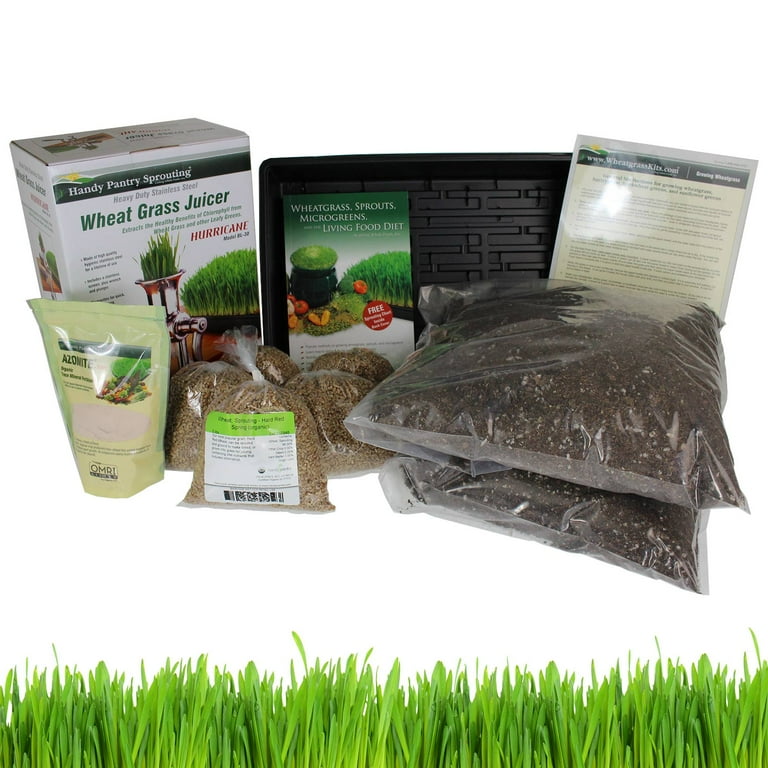This color image is a composite of two photographs set against a white background. The top section showcases a variety of gardening and lawn care products, while the bottom section features a close-up of lush, green lawn grass.

In the upper part of the image, on the left side, there's a prominent white box labeled "Handy Pantry Sprouting Wheat Grass Juicer" with an additional phrase "Hurricane Heavy Duty Stainless Steel" written in gray. This box also features an image of grass growing in a planter. In front of this box, there is a green pouch with unreadable text. Adjacent to the green pouch, several smaller clear plastic bags are displayed, each containing brown seeds and adorned with an unreadable white and green label.

To the right, further in the foreground, stand two bags of gardening soil. Behind these bags, there is a black plastic tray labeled "Wheat Grass Sprouts Microgreens Living Food Diet." Beyond the tray and the soil bags, a small placard with white and black print, likely containing instructions or a care chart, is visible though not legible.

The unified white background and the vibrant green grass at the bottom create a stark contrast, emphasizing the connection between the supplies and their application.